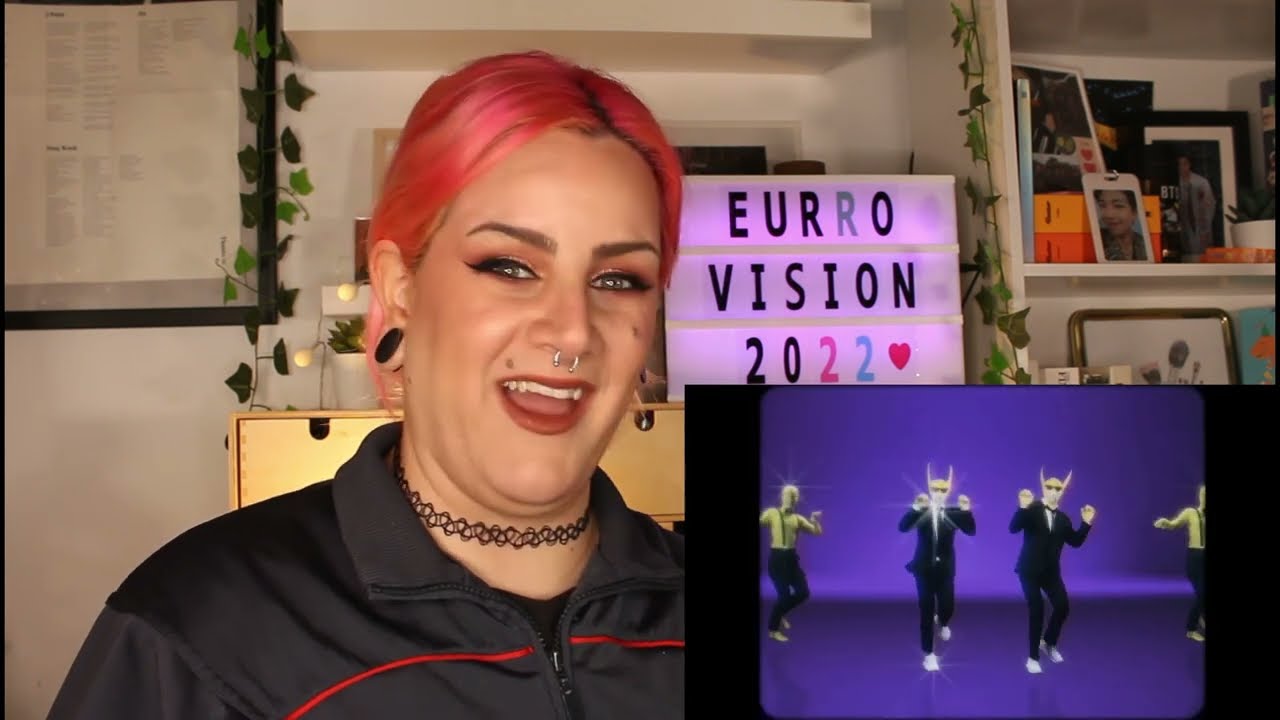In this screen capture of a reaction video, a Caucasian woman with vibrant pink hair, round black gauged earrings, and a silver nose ring is seen laughing. She wears a black zip-up jacket accented with red lines and a black choker. Her background is a decorated room with shelves, picture frames, vines, and a light-up sign that reads "Eurovision 2022" with a pink and blue color scheme. A smaller picture-in-picture in the lower right corner shows the video she's reacting to: a quirky dance performance with four individuals. The two central figures wear black suit coats, yellow masks with long ears, and glasses, giving them a cat-like appearance. Behind them, two other dancers in white shirts, black suspenders, and black pants mirror cat-like gestures. The background for this dance appears purple, enhancing the surreal, whimsical effect.